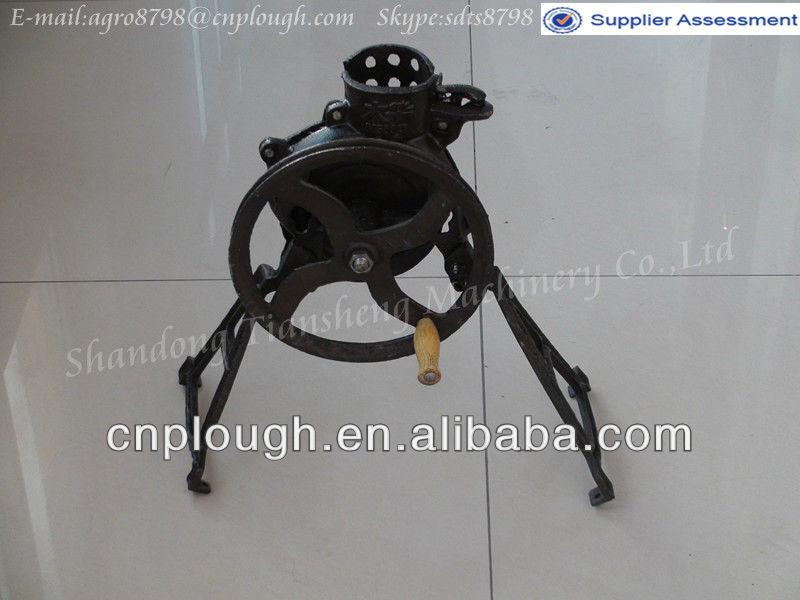The image depicts a black, antique-style grinder positioned upright on a white or gray tiled floor. The grinder features a large spinning wheel with a wooden handle, a cup at the top, and two base legs for stability. Above the product, text reads "email agro8798 at cnplough.com" and "Skype sdts8798." In the upper-right corner, a small badge states "supplier assessment." A faint watermark across the image displays "Shandong Tiansheng Machinery Co. Ltd," and below the grinder, "cnplough.en.alibaba.com" is visible. The overall photograph appears to be a product image for a website, capturing the old-fashioned iron machinery in a straightforward, upright manner. The dominant colors are black for the grinder and white or gray for the floor tiles.